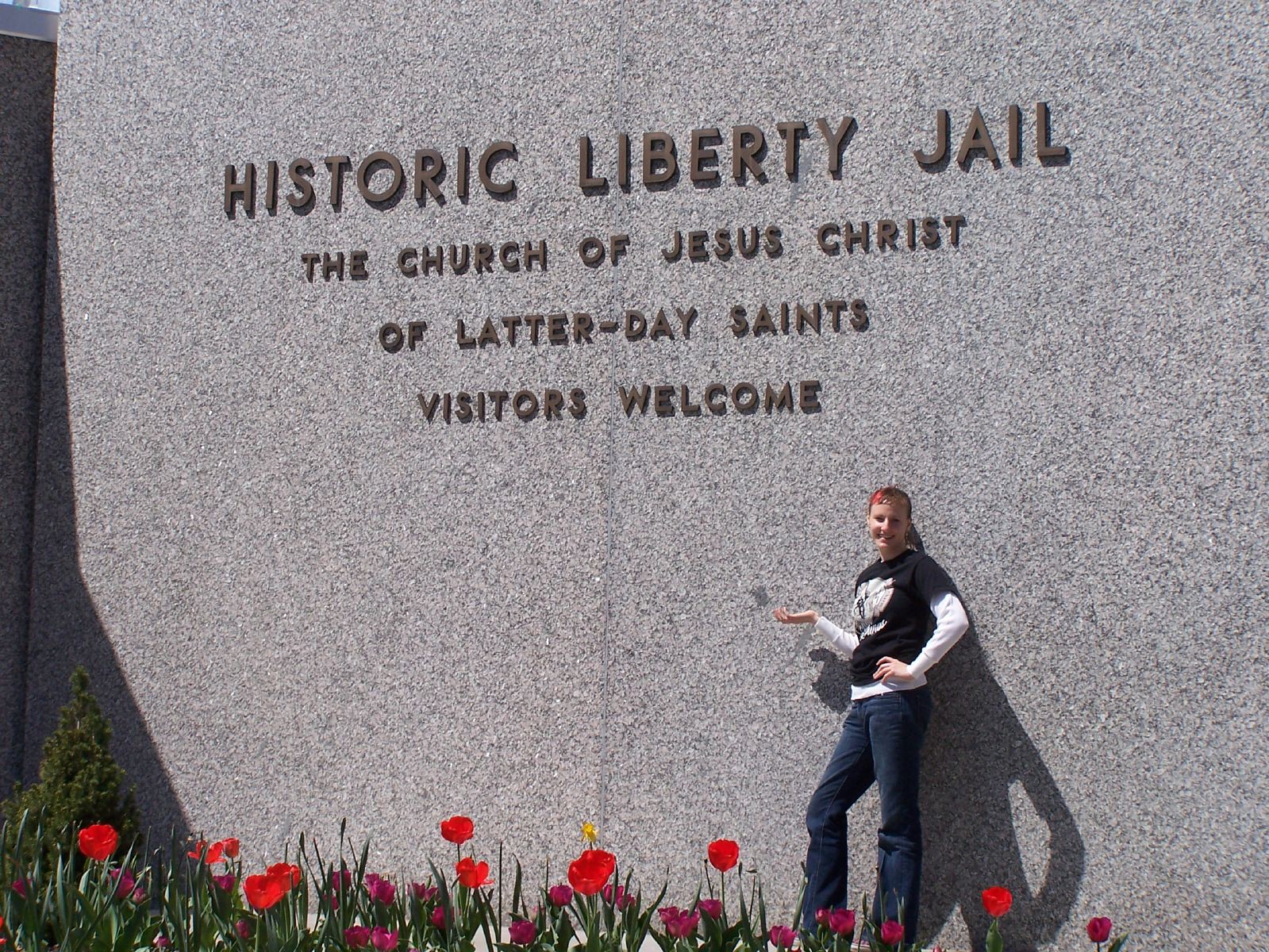The image captures a detailed scene set in front of a massive gray cement wall, which is prominently inscribed with dark gray extruded lettering. The text, in all capital letters, reads: "Historic Liberty Jail" at the top line, followed by "The Church of Jesus Christ of Latter-day Saints" and "Visitors welcome." Below these inscriptions, a variety of flowers — red and purple, with green stems — bloom vibrantly at the base of the wall, along with a small, shadow-clad pine tree to the bottom left. A young person with a mix of reddish and brownish hair stands confidently in front of the wall. They are dressed in a black t-shirt with a white graphic over a long-sleeved white shirt and blue jeans, posing with their left hand on their hip and their right arm extended forward. The sunlight casts a distinct shadow of their figure upon the cement wall, adding depth and contrast to the outdoor scene.